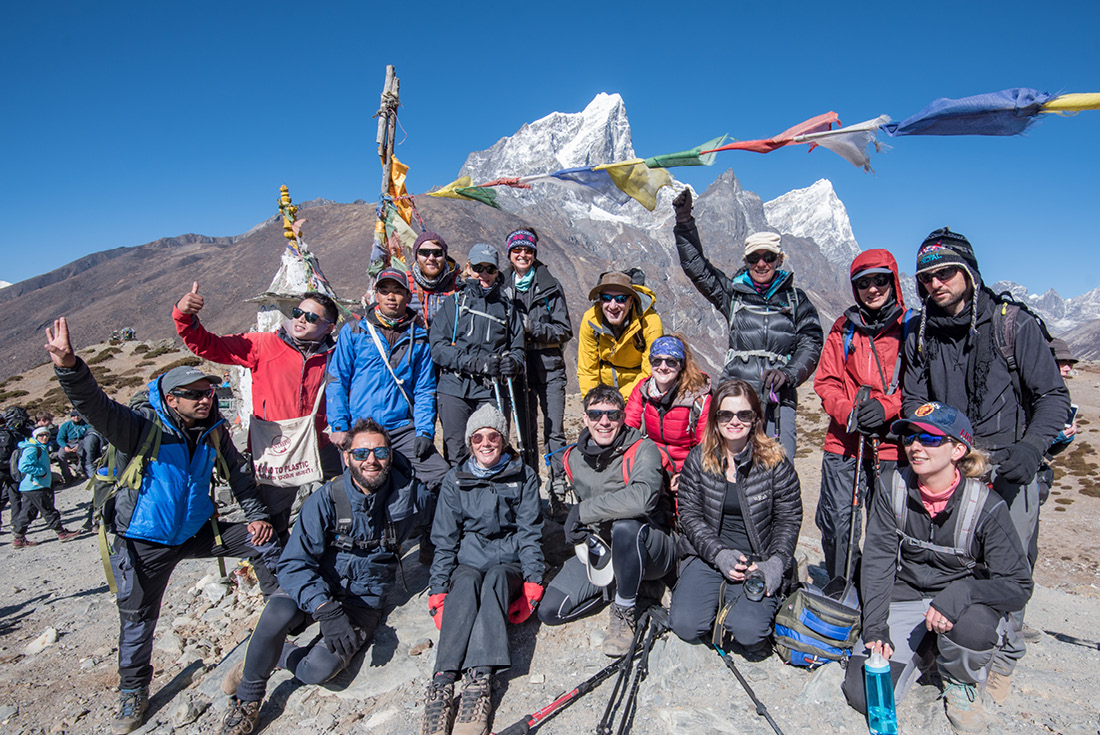The photograph is a vibrant snapshot of 16 jubilant hikers who have reached their mountain summit, with a majestic, snow-capped mountain and an expansive, cloudless blue sky serving as a stunning backdrop. The group, which consists of both men and women, is dressed in a variety of cold-weather hiking gear, including wind jackets, winter jackets, hats, bandanas, and sunglasses—with only one person not wearing glasses, possibly a native guide in a blue coat. All the hikers are smiling at the camera, exuding accomplishment and joy. Some hikers are giving thumbs up, while one man prominently holds up four fingers, perhaps marking his fourth ascent. In the foreground, various hiking paraphernalia like water bottles and poles can be seen. Above the group, colorful flags flutter from a flagpole, adding to the celebratory atmosphere and hinting at a possible base camp, reminiscent of Everest.